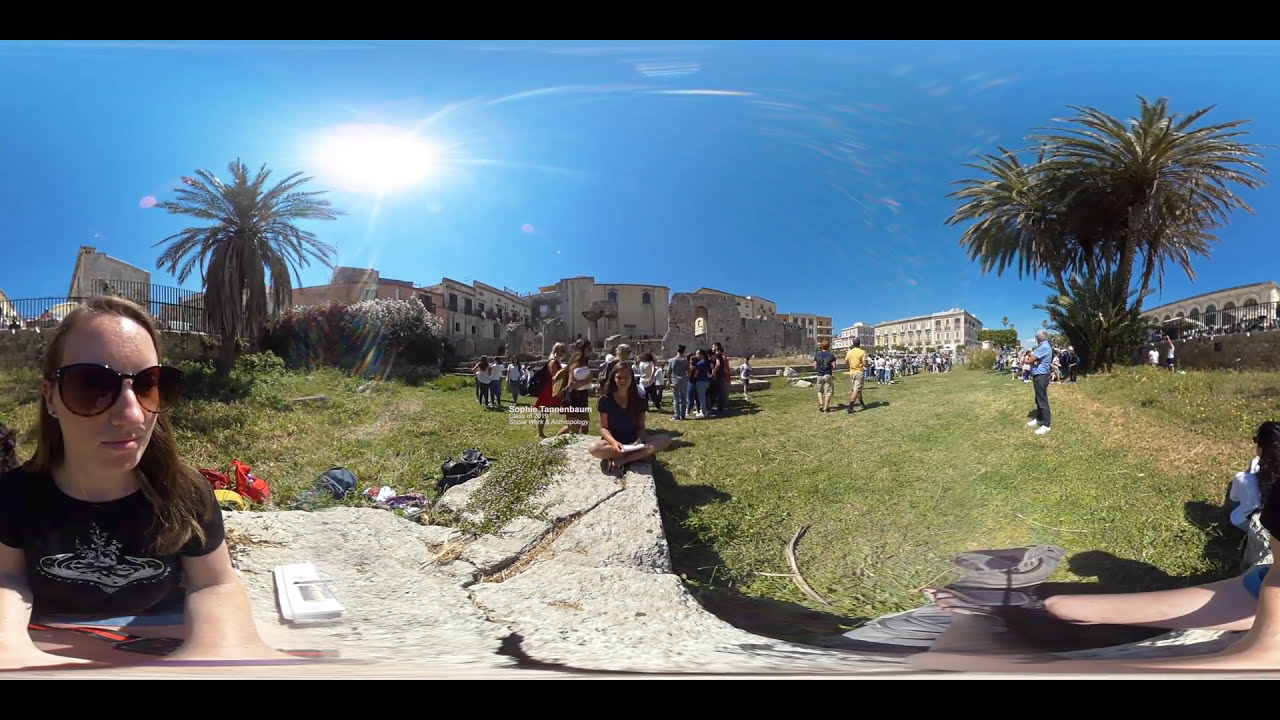The image captures an outdoor gathering beneath a bright, clear blue sky. Prominently featured at the very bottom left is an unsmiling woman with long brown hair and sunglasses, wearing a black t-shirt. She appears to be standing on a rock walkway with a backdrop of lush green grass. Behind her, various people are scattered across the scene, including some standing near palm trees to the right and a couple of individuals in white clothing, with colorful bags on the ground nearby. The middle of the image is dominated by a text reading "Sophie Tannenbaum, class of 2019, social work in anthropology," positioned next to a woman seated on a cracked stone ledge, possibly Sophie. She has her legs crossed in a relaxed manner. Surrounding the central characters are additional people: a man in a light blue shirt and dark pants standing with his arms crossed, near him two men walk away—one in a blue shirt and tan pants, the other in a yellow shirt and tan pants. The background is filled with palm trees, flowers over a fence, and older-looking buildings in shades of gray, tan, and white. The bright sunshine illuminates the lively yet serene atmosphere, possibly indicative of a school or college event.